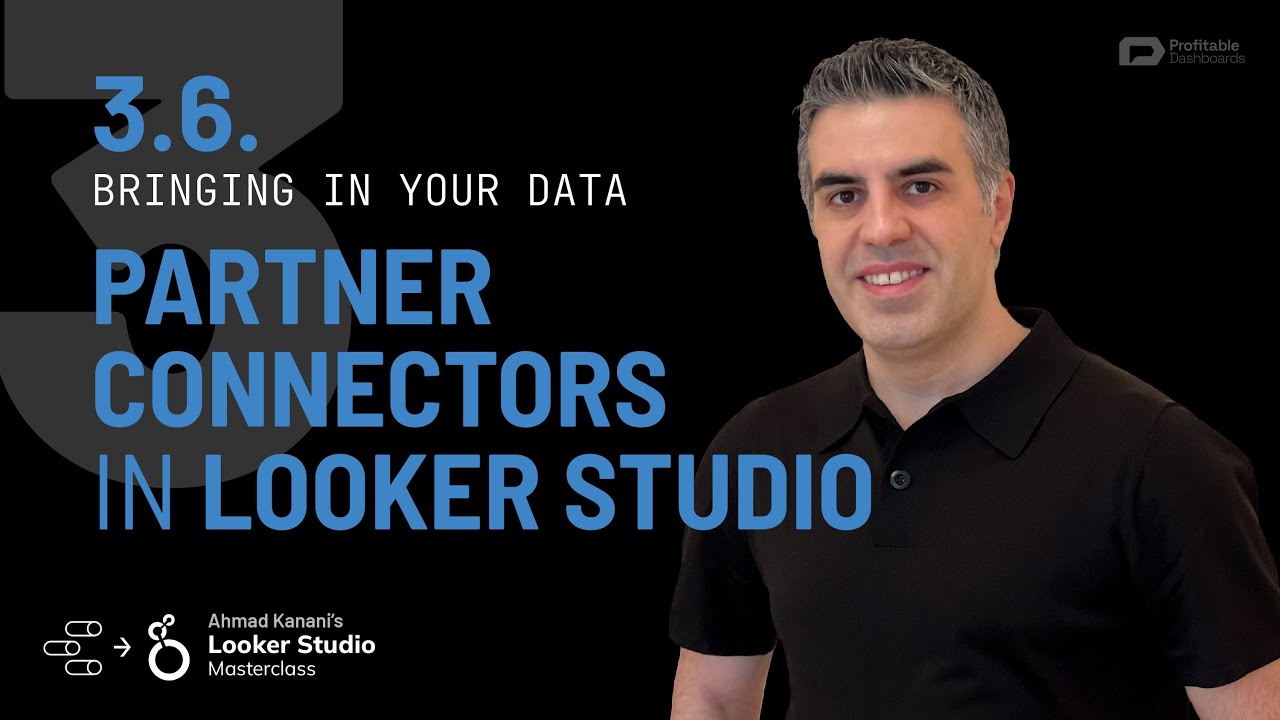The image features a rectangular screen in landscape orientation with a predominantly black background. In the upper left quadrant, a large numeral "3" in gray subtly blends into the background. On the right side, a portrait of a man is prominently displayed from the chest up. He is dressed in a black polo shirt, exposing his arms up to the elbows. He has short, salt-and-pepper hair, neatly combed away from his face, and exhibits dark eyebrows and dark eyes. His expression is pleasant, with his mouth slightly open, revealing his teeth. 

In the upper right corner of the image, a small icon accompanied by the words "ProfitAble Dashboards" is visible. At the top left of the screen, large blue text reads "3.6". Directly below, in white capital letters, the text states "BRINGING IN YOUR DATA". Further below, bold and capitalized blue text is divided into three lines: "PARTNER", "CONNECTORS", and "IN LOOKER STUDIO". At the bottom left corner of the screen, three horizontal cylinders drawn in white are followed by a right arrow and three interlocking white rings. To the right of these symbols, the text reads "Ahmad Kanani's Looker Studio Masterclass".